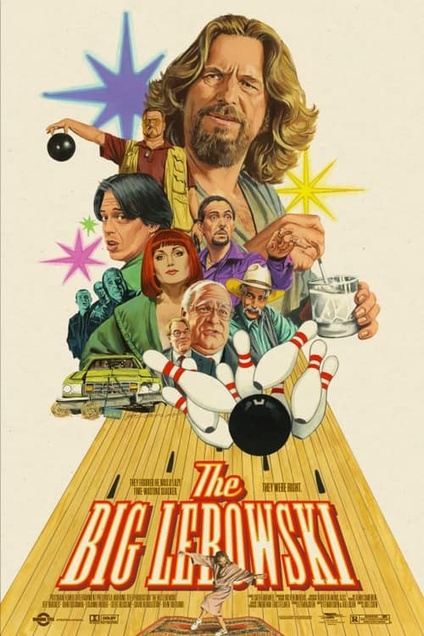This is a retro-styled movie poster for "The Big Lebowski" set against a white background, reminiscent of a 90s artistic vibe. It prominently features the movie title "The Big Lebowski" in large white text with a red outline at the bottom, positioned at the forefront of a bowling alley lane. A bowling ball is captured mid-motion, striking pins that scatter along the lane. Above this dynamic scene, the poster transitions into a collage of the film's diverse characters. Central to the image is a middle-aged man with shoulder-length, wavy dirty blonde hair and a goatee beard, portrayed with an artistic rendering at the top. Surrounding him are various other figures, including a woman with short red hair in a green jacket, a hefty man holding a bowling ball while wearing glasses, a red shirt, and a yellow vest, and a man in a green outfit. Additionally, there's a man depicted with black facial hair and a purple shirt, a yellow car among the characters, and an assortment of other figures, including a cowboy hat-wearing individual and a fisherman jacket-clad man. Intermingled with these characters are vibrant, light colors contributing to the overall lively and engaging feel of the poster.